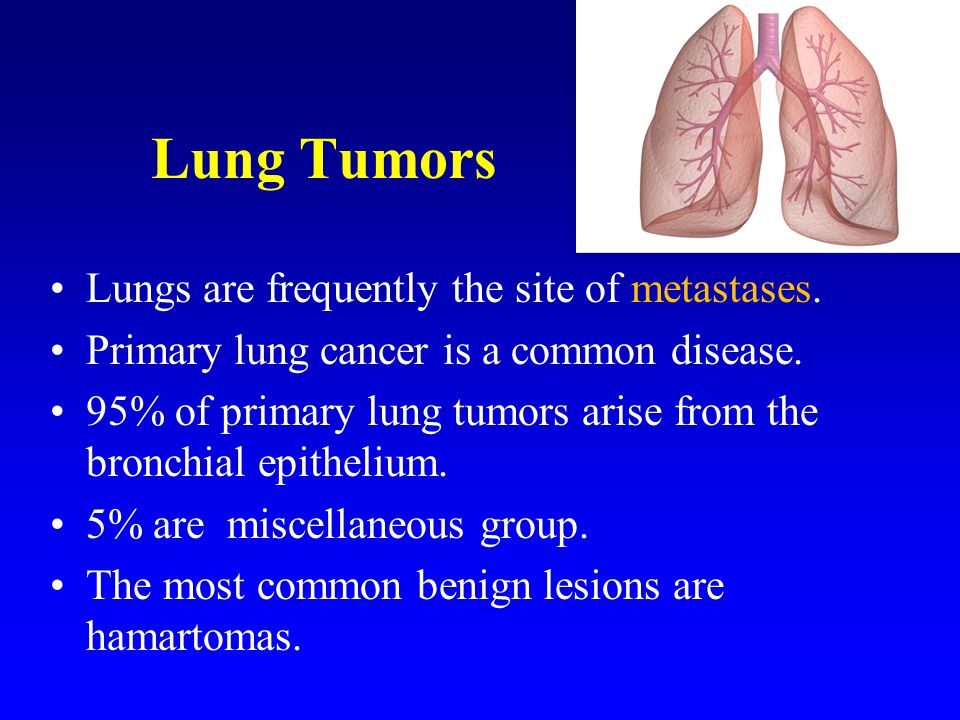The image is a detailed screenshot of an educational medical slide about lung tumors with a distinct blue theme. Dominating the top right corner is a detailed diagram of human lungs, complete with ventricles, passageways, and airways. The title "Lung Tumors" is prominently displayed in yellow at the top. The content includes several bullet points in white text on a blue gradient background. The bullet points highlight key information: lungs are frequently the site of metastases, primary lung cancer is a common disease, 95% of primary lung tumors originate from the bronchial epithelium, 5% fall into a miscellaneous group, and the most common benign lesions are hamartomas. Overall, the slide serves as a comprehensive educational resource on lung tumors and their causes.